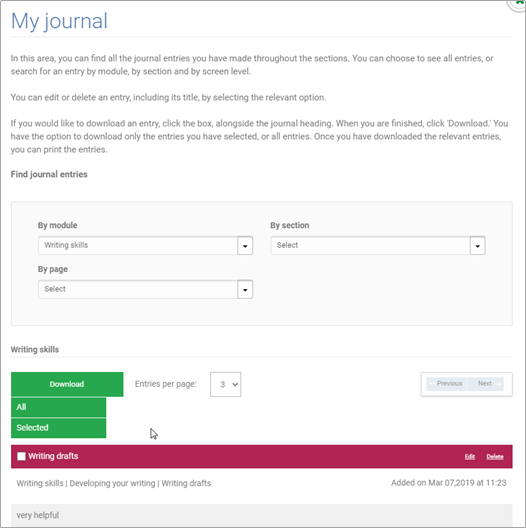"Explore comprehensive journal entry management in this detailed guide. On this screen, users can view all journal entries or search by specific parameters including module, section, and screen level. Enhance productivity by editing or deleting entries through easy selection options. To download an entry, simply click the checkbox next to the journal heading and initiate the download process. Users can choose to download selected entries or the entire list. Once downloaded, entries are readily available for printing.

On the interface, the 'Find Journal Entries' section includes filters by module such as Writing Skills, selectable from a drop-down menu. Further refine your search by section and page, also available via drop-down menus. The interface highlights Writing Skills modules in green, with action buttons such as 'Download' (green) for downloading all or selected entries, and options to select entries per page.

Navigational buttons for 'Previous' and 'Next' are located to the right. Below these, the purple bar titled 'Writing Drafts' indicates the status of drafts. Entries include descriptive details like title, module, sections of 'Writing Skills,' and specifics such as 'Developing and Writing,' and timestamps like 'Added on March 7, 2019, at 11:23.' User feedback can also be viewed, marked as 'Very Helpful.' To the far right, you will see an 'X' for closing the window.

This user-friendly platform ensures efficient journal entry management and enhances writing skill development through structured organization and detailed entry information."